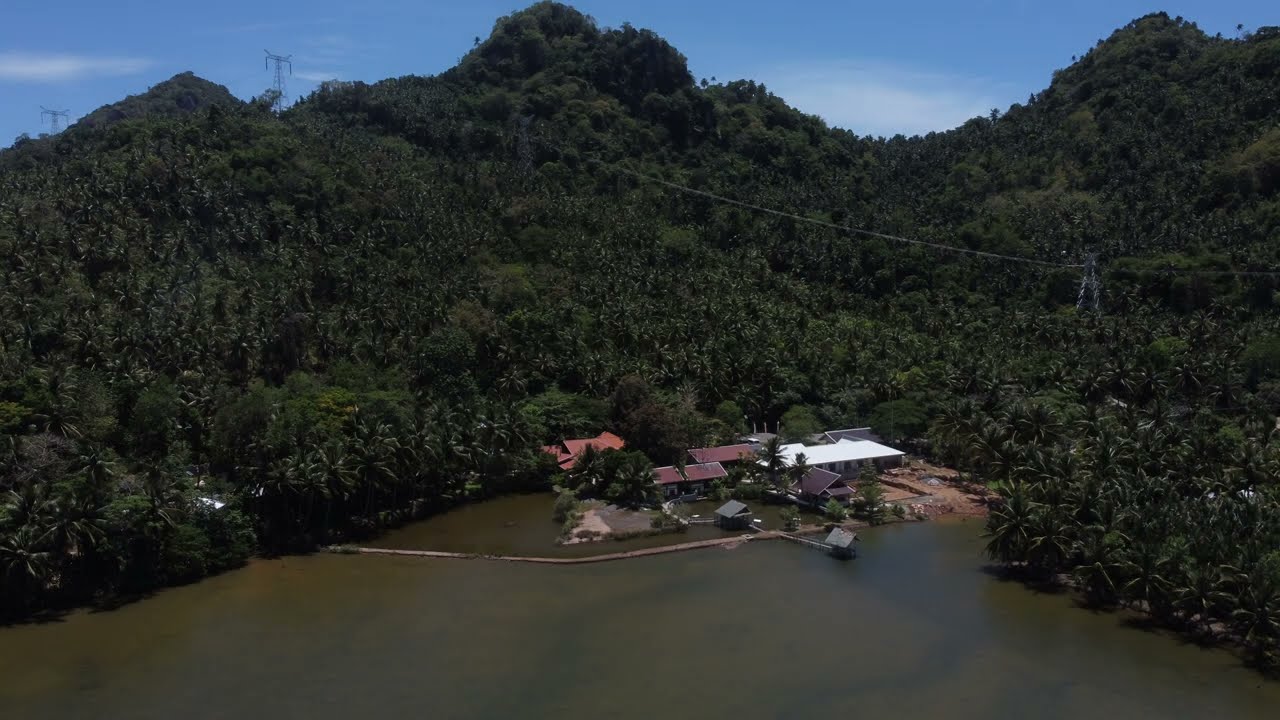The image depicts a serene bay area surrounded by dense tropical greenery and rolling hills. At the center of the photograph, nestled near the water's edge, lies a small compound featuring around five buildings, each with roofs in varying shades of red, white, and gray. The compound includes homes that are connected together, encircled by trees, and bordered by brownish-green water. A cement bridge and a long dock extend into the water, indicating some small boat activity. The lush hills behind the compound are blanketed with a variety of tropical plants and trees, including palm trees, giving the area a vibrant green appearance. The blue sky above is clear, adding to the peaceful, daytime setting. Running through the hills, from the right-hand side up to the upper left-hand side, are some gray power lines, subtly blending into the natural landscape.